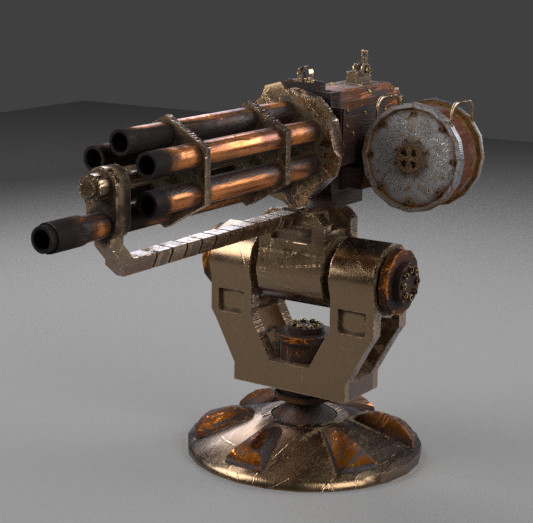The image depicts a bronze or copper sculpture that intricately resembles an old-fashioned, rotary machine gun. The sculpture features a flat, circular base and stands less than a foot high, resting on a gray countertop against a shadowy, darker gray wall. Central to the sculpture is a component resembling a belt buckle with a screw and bolt through the middle. The upper part showcases six openings akin to gun barrels and includes adjacent copper rods. On the right side, there's an element that might be a scope, evocative of a spool with holes, while the left side suggests a slot for bullets or casings. The piece, imbued with a touch of rust, combines elements of a real weapon with artistic flair, blending bronze and possibly silver metals.